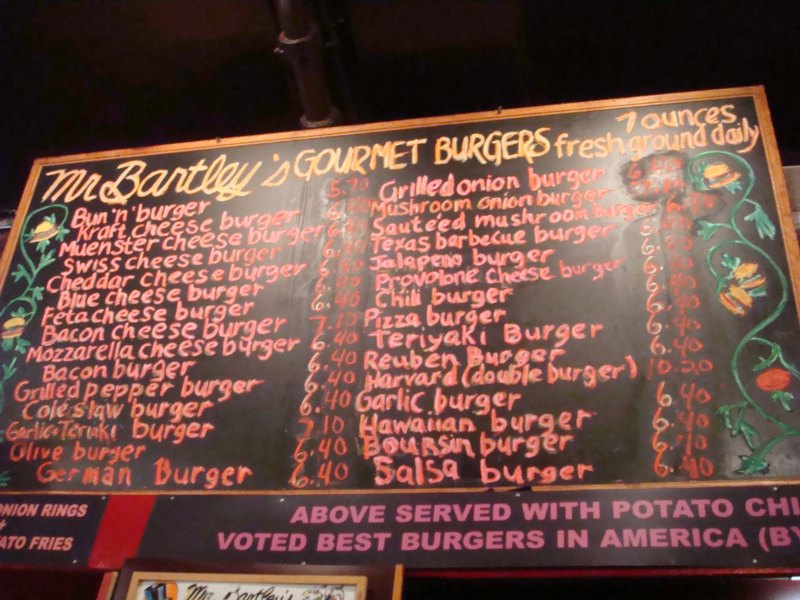The image depicts a rustic restaurant menu designed to resemble a black chalkboard. At the top, in elegant cursive and light orange text, the title "Mr. Bentley's Gourmet Burgers" is prominently displayed. Beneath the title, an inscription reads, "seven ounces fresh ground daily," in the same light orange color but in standard lettering.

On the left-hand side of the menu, a list of burgers is presented in neat, sequential order:
- Bun and Burger
- Kraft Cheeseburger
- Munster Cheeseburger
- Swiss Cheeseburger
- Blue Cheeseburger
- Feta Cheeseburger
- Bacon Cheeseburger
- Mozzarella Cheeseburger
- Bacon Burger
- Grilled Pepper Burger
- Coleslaw Burger
- Garlic and Teriyaki Burger
- Olive Burger
- German Burger

Each burger name is written in an orange-pink hue, and prices are listed to their right. Accompanying this list is a decorative floral design on the left side, featuring green foliage and two yellow bell-shaped flowers.

On the right-hand side, another series of burger options, written in the same orange-pink text, includes:
- Grilled Onion Burger
- Mushroom Onion Burger
- Sauteed Mushroom Burger
- Texas Barbecue Burger
- Jalapeno Burger
- Provolone Cheeseburger
- Chili Burger
- Pizza Burger
- Teriyaki Burger
- Reuben Burger (Harvard in parentheses)
- Double Burger
- Garlic Burger
- Hawaiian Burger
- Boursin Burger (spelled out)
- Salsa Burger

Mirroring the left side, a similar floral pattern adorns the right side of the menu. Below this list, in purple text, a statement reads: "Above served with potato chips. Voted best burgers in America." Adjacent to this declaration is a red rectangle on the left.

The entire menu is framed in a light brown wooden border, providing a rustic touch. The background color of the menu is black, creating a striking contrast with the colorful text and decorative elements.